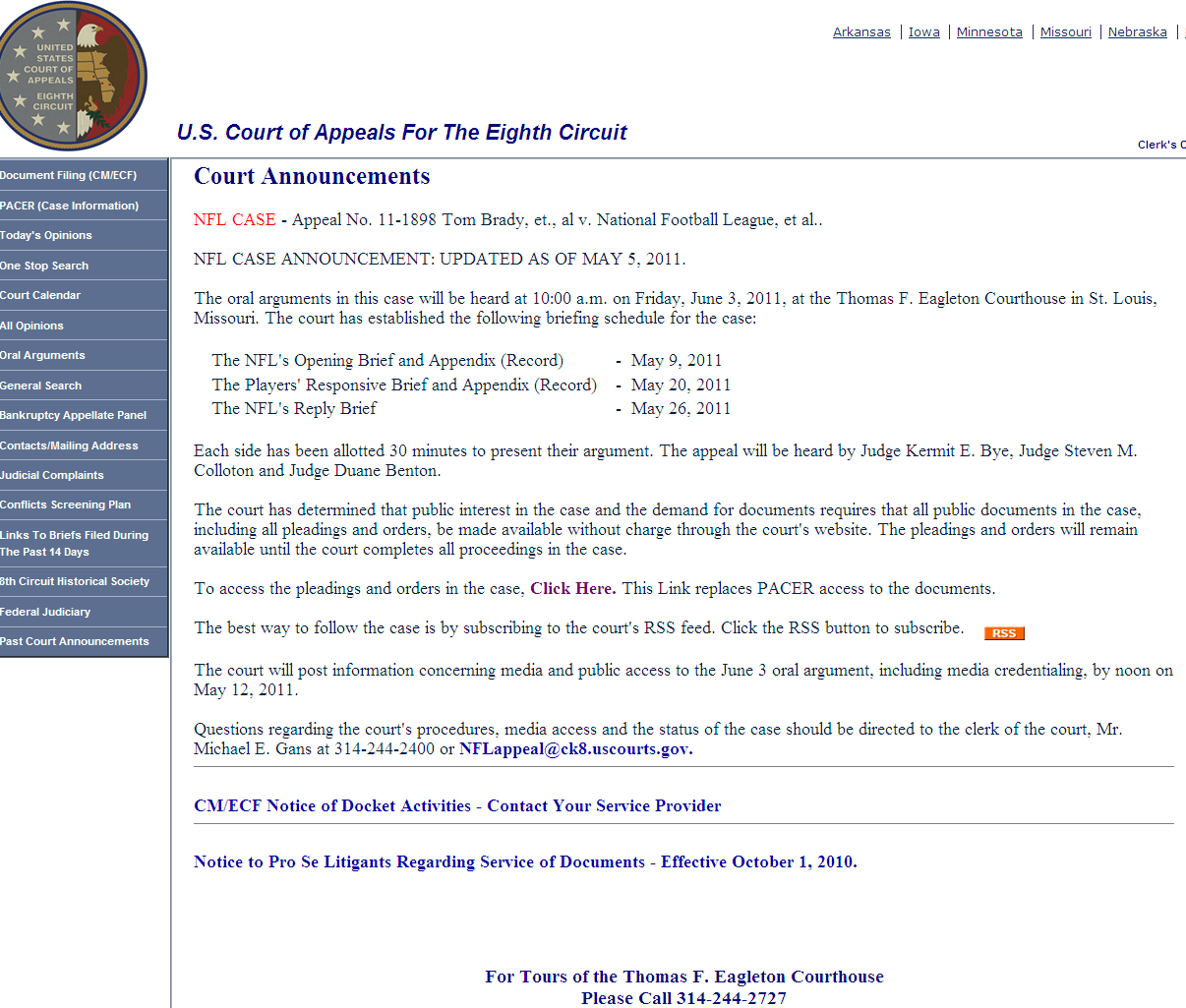This image features a well-structured webpage from the United States Court of Appeals for the 8th Circuit, set against a predominantly white background. In the top left corner, there is a detailed circular emblem with the left half in gray adorned with stars around the outer edge. Inside, "United States Court of Appeals, 8th Circuit" is inscribed in white. The right half of the circle contains a detailed depiction of an eagle with its head turned to the right against a vivid red background. This emblem is surrounded by three borders: purple, brown, and a darker brown.

Just below, two inches from the left margin and occupying approximately two-thirds of the page vertically, there is a blue section featuring white text. This section hosts 14 clickable tabs for navigation. Adjacent to the eagle, and slightly downwards, "U.S. Court of Appeals for the 8th Circuit" is displayed prominently in dark blue, beneath which a horizontal blue line spans the width of the page. 

In the top left corner, a list of states—Nebraska, Missouri, Minnesota, Iowa, and Arkansas—is printed in blue, each underlined and separated by small dividing lines. Just below, on the right, "Clerks See" is noted. Beneath the "U.S. Court of Appeals" header, bold "Court Announcements" appears, succeeded by "An NFL Case" in red, detailing information on the Tom Brady case with the National Football League. Subsequent black text provides update information, followed by several lines of details, dates, and events, maintaining a consistent and informative structure.

Towards the bottom, in purple letters, contact information is specified alongside the dates when documents were filed. Centrally located at the footer, there is a note about tours of the Thomas F. Eagleton Courthouse, accompanied by a phone number for enquiries.